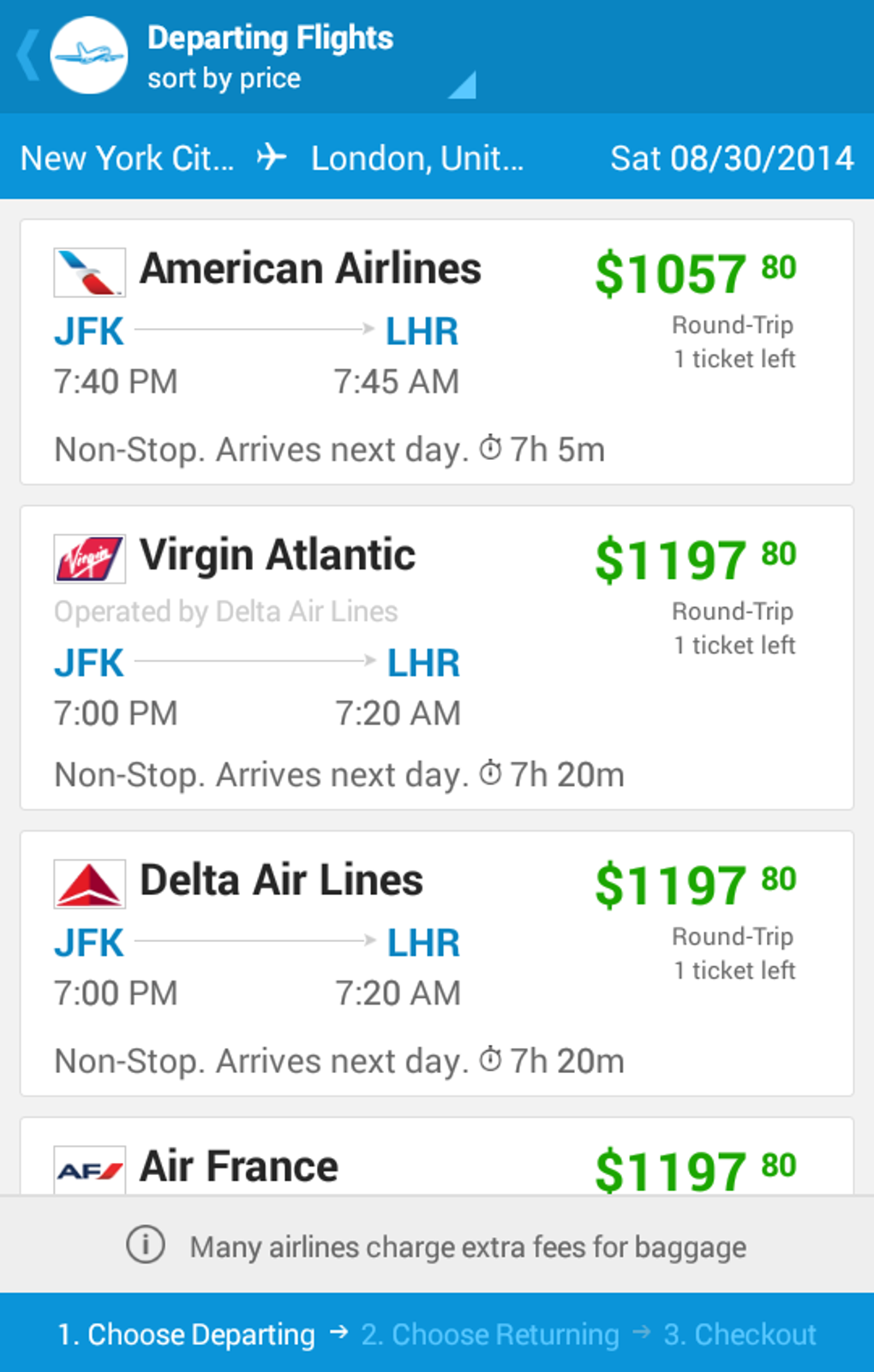The image depicts a detailed digital display for departing flights. At the top, there's a title "Departing Flights," accompanied by a white circle featuring an icon of a blue airplane. The display allows sorting by price. 

The schedule lists several flights to London from New York City on Saturday, August 30, 2014:

1. **American Airlines**  
   - Route: JFK to LHR  
   - Price: $10,057.80 round-trip
   - Availability: 1 ticket left
   - Flight Type: Non-stop
   - Duration: 7 hours 5 minutes
   - Arrival: Next day

2. **Virgin Atlantic** (operated by Delta Air Lines)  
   - Route: JFK to LHR  
   - Price: $1,197.80 round-trip
   - Availability: 1 ticket left
   - Flight Type: Non-stop

3. **Delta Air Lines**  
   - Route: JFK to LHR  
   - Price: $1,197.80 round-trip
   - Availability: 1 ticket left
   - Flight Type: Non-stop
   - Duration: 7 hours 20 minutes
   - Arrival: Next day

4. **Air France**   
   - Route: (Details partially cut off)
   - Price: $1,197.80 round-trip

Below the main flight listings, there is a gray section containing a circle with an "i" icon, accompanied by the note: "Many airlines will charge extra fees for baggage."

At the bottom, a blue navigation strip is displayed, guiding the user through the booking process with steps: 
1. Choosing Departing (with an arrow)
2. Choosing Returning (with an arrow)
3. Checkout